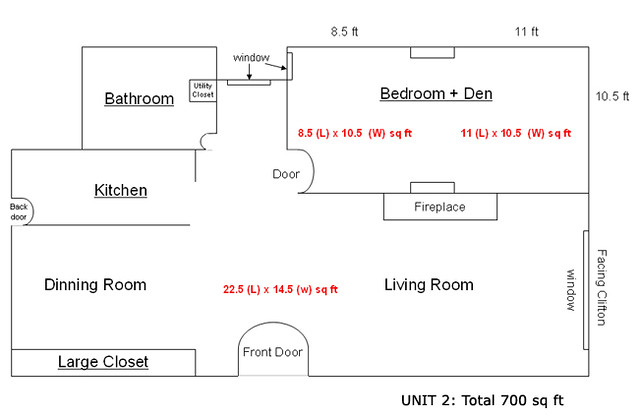This detailed schematic drawing depicts a unique residential layout where every line is of uniform thickness. The residence includes various rooms, such as two bedrooms, a den, a kitchen, a dining room, a living room, a large closet, a utility closet, and features both front and back doors. Additionally, a cozy fireplace is present.

The diagram emphasizes certain rooms—namely the kitchen, bathroom, bedroom, den, and large closet—by underlining them, while other labels remain plain. Red font annotations provide specific dimensions for the living room, dining room area, as well as for the combination bedroom and den. These dimensions include 8.5 feet by 10.5 feet, and 11 feet by 10.5 feet, suggesting the total area of the bedroom and den combined. The total living area of the residence is noted as 700 square feet, hinting that it might be a compact apartment despite the inclusion of a back door. The front door faces Clifton, adding a point of interest about its orientation.